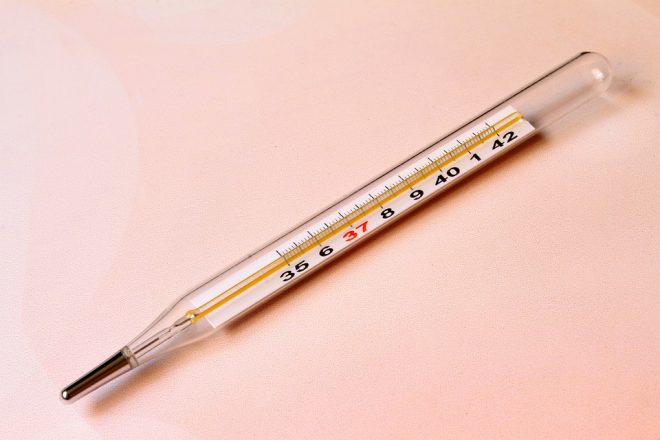The image depicts a photograph of a glass thermometer placed on a solid pink background, possibly a table or countertop. The thermometer has a metal tip and features several marked lines accompanied by numbers inside the glass tube. The sequence of numbers, which are read from left to right, are 35, 36, 37 (in red), 38, 39, 40, 41, and 42. This sequence might suggest it is a tool for measuring temperature, although the numbers appear unconventional for a standard human thermometer.